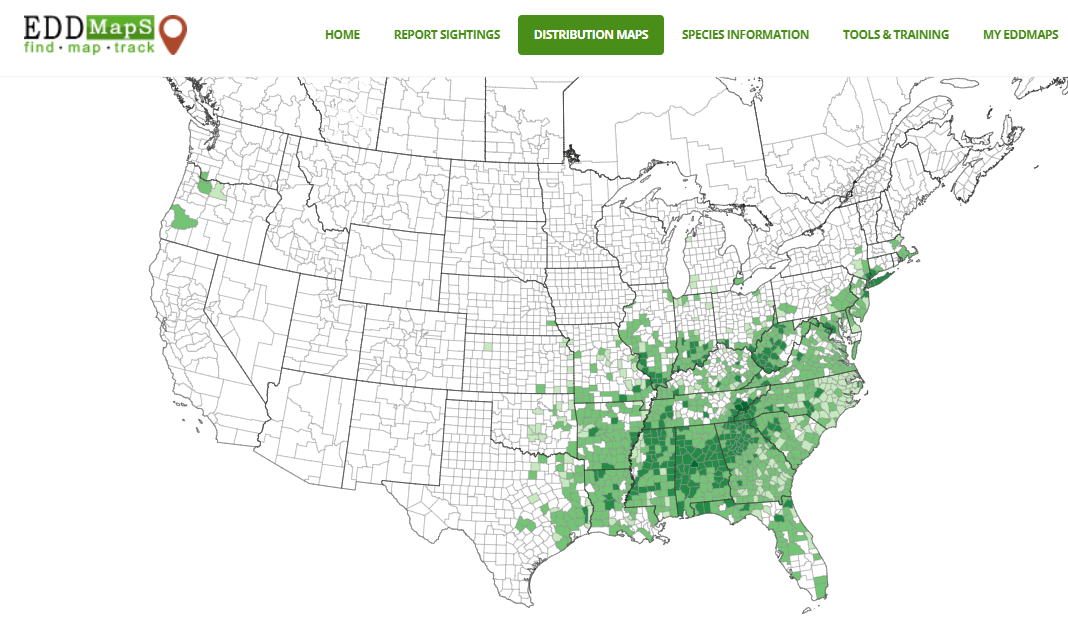This image is a detailed distribution map of the United States, specifically provided by EDD Maps. The map primarily highlights regions of the southern United States, showing various concentrations of green dots that represent specific data distributions. The heaviest green areas are in Mississippi and Alabama, with coverage extending from East Texas up to Maryland and West Virginia, then westward to Indiana, and down to Florida. The map's background is a gray and white outline of the United States, and it features a header bar with several clickable buttons, including Home, Report Sightings, Distribution Maps, Species Information, Tools and Training, and My EDD Maps. A red button with a white center is located in the left-hand corner of this header. The map visually differentiates regions with patterns in light and dark green, indicating varying densities of the tracked parameter across the southern states like Georgia, Alabama, Mississippi, Arkansas, Louisiana, Texas, Missouri, Kentucky, Indiana, West Virginia, Virginia, North and South Carolina, and Florida.